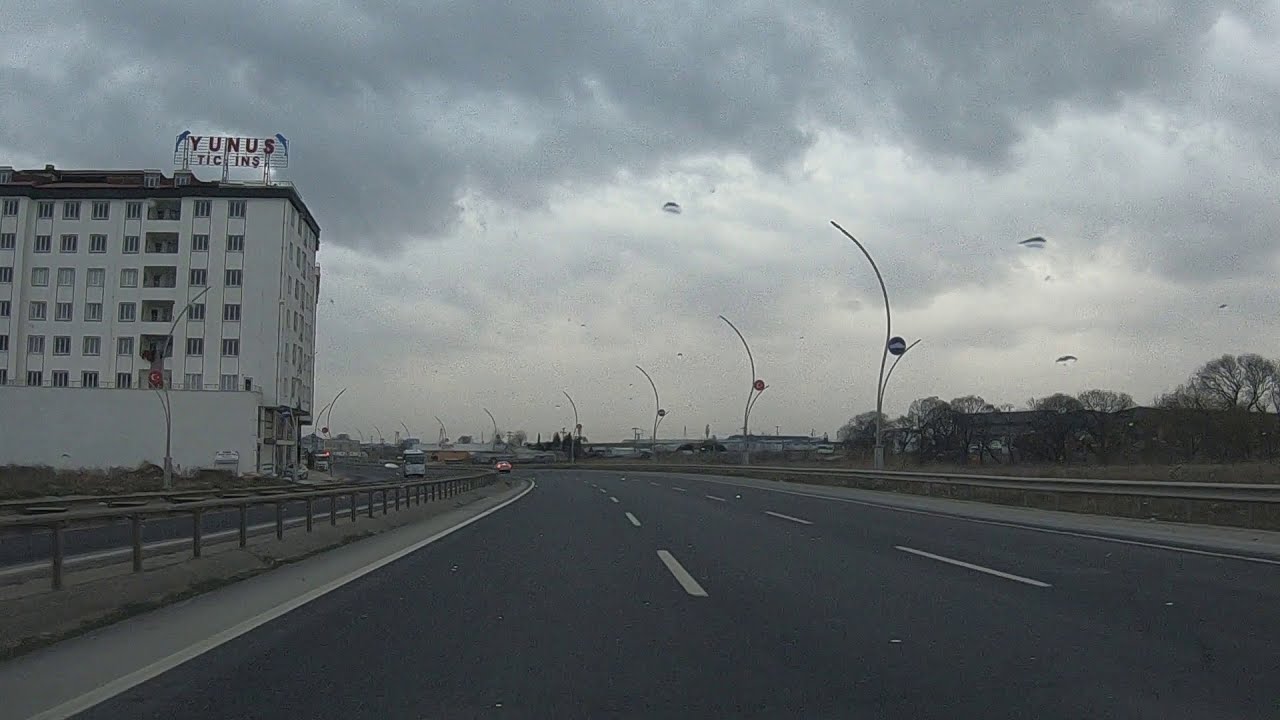The image depicts a three-lane highway on the outskirts of a city, viewed from the leftmost lane. The grayish roadway curves slightly to the left in the distance, showcasing light gray stripes. There are a few cars in the distance with minimal traffic on the road. Streetlights arch over both sides of the highway, more prominent on the right. A tall, light gray building labeled "Y-U-N-U-S" and "T-I-C-I-N-S" stands on the left side, featuring windows facing the road. On the right side, beyond the guardrail, lies a grassy area leading to a cluster of leafless trees, indicating a fall or winter season. The sky is overcast with dark clouds, and faint water droplets are visible on the lens, adding to the stormy ambiance.